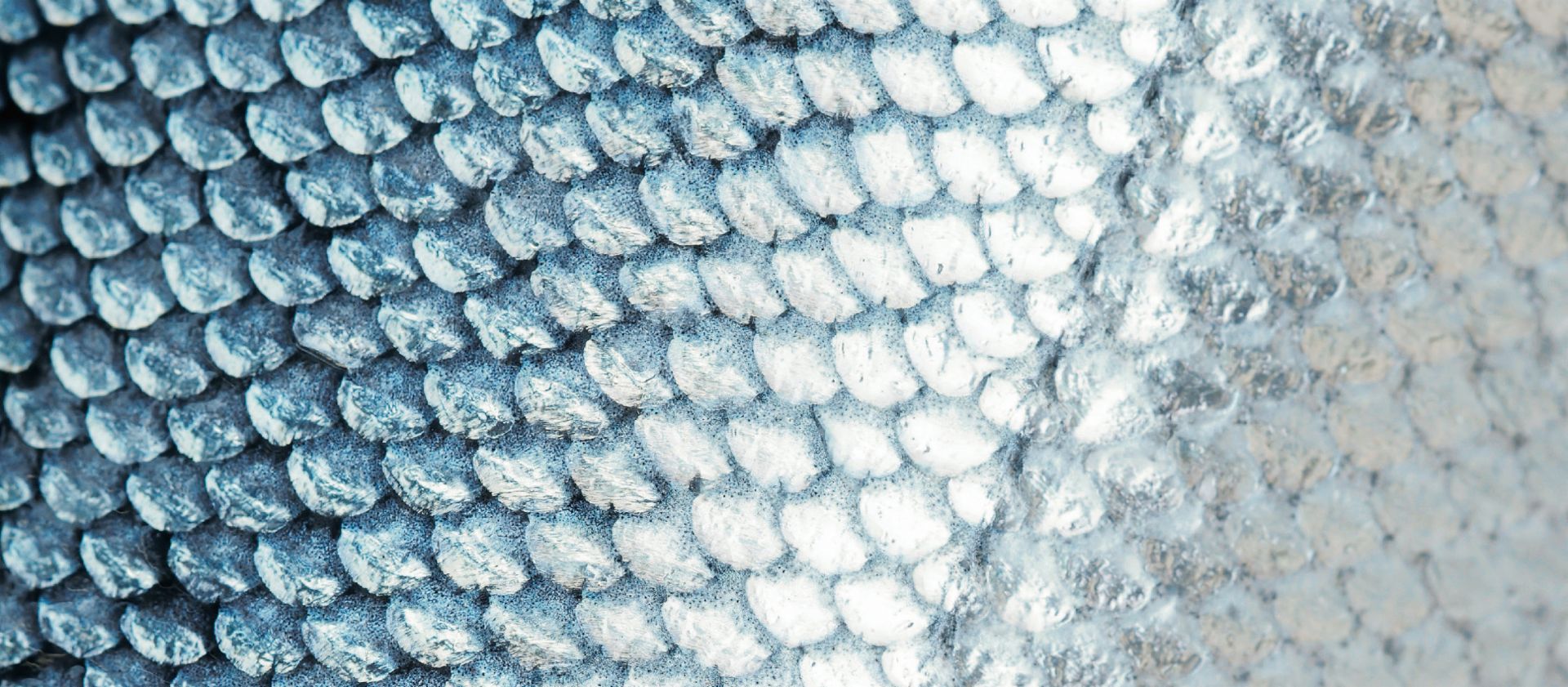The image captures an extreme close-up of scales, likely from a fish or possibly a lizard, rendered in exquisite detail. The scales are predominantly silver, transitioning into a metallic blue on the left side. A strong highlight in the center of the image accentuates the texture and raised nature of the scales, making them appear more three-dimensional. The light source also creates a gradient effect, with the brightness fading into darker shades towards the edges. On the right side, the scales become slightly blurred, possibly out of focus, adding depth to the photograph. The scales appear dry, suggesting that the creature might no longer be alive. The intricate detailing, with black outlines between the scales on the left, makes for a mesmerizing and beautifully detailed close-up image.